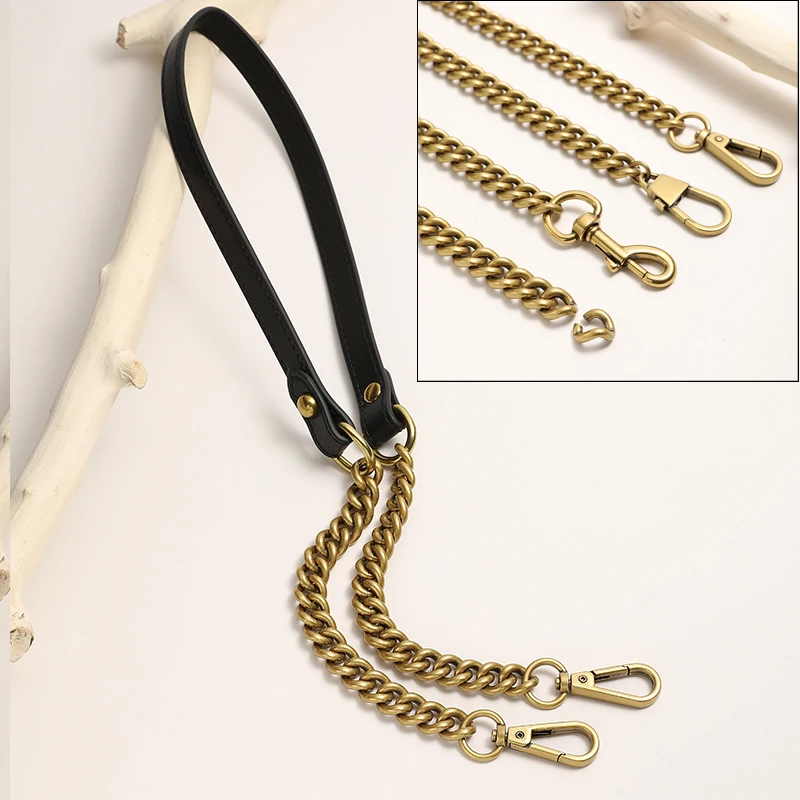The photograph captures a detailed display of a black leather strap with gold chain ends. The strap, appearing like a purse handle, features rivets and alligator clips at each end and rests against a smooth, white tree branch on a pale pinkish-gray background. An inset image within the main picture showcases four additional gold chains, each with varying styles of clips, including an open oval-shaped clip, a button clip, and a snap-on clip. One of the chains in the inset is broken, with a missing link visible at the end.